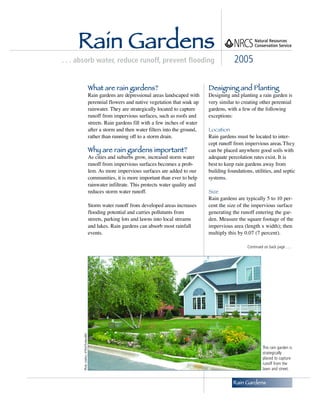This infographic from the NRCS (Natural Resources Conservation Service) titled "Rain Gardens: Absorb Water, Reduce Runoff, Prevent Flooding" offers detailed information on rain gardens in a layout designed to educate readers. The infographic, dated 2005, highlights the benefits of rain gardens at the top with the key goals listed: absorption of water, reduction of runoff, and prevention of flooding. 

The main body of the infographic is divided into sections by a thin black line and features six paragraphs of text under three primary blue-inked headings. The first section, "What are Rain Gardens?" provides a focused definition of rain gardens. This is followed by, "Why are Rain Gardens Important?" which comprises two paragraphs detailing their significance. The final section is titled "Designing and Planting," which consists of three paragraphs that guide readers on how to design and plant a rain garden and includes insets on choosing location and site specifics.

Below the textual information, the infographic features an inset image of a residential front yard showcasing a rain garden. This garden appears slightly recessed, filled with various wild plants, and is bordered by a lush green lawn. A picturesque farmhouse-style blue house serves as the backdrop, with a manicured tree to the left, enhancing the visual example of a rain garden's potential integration into a typical home landscape.